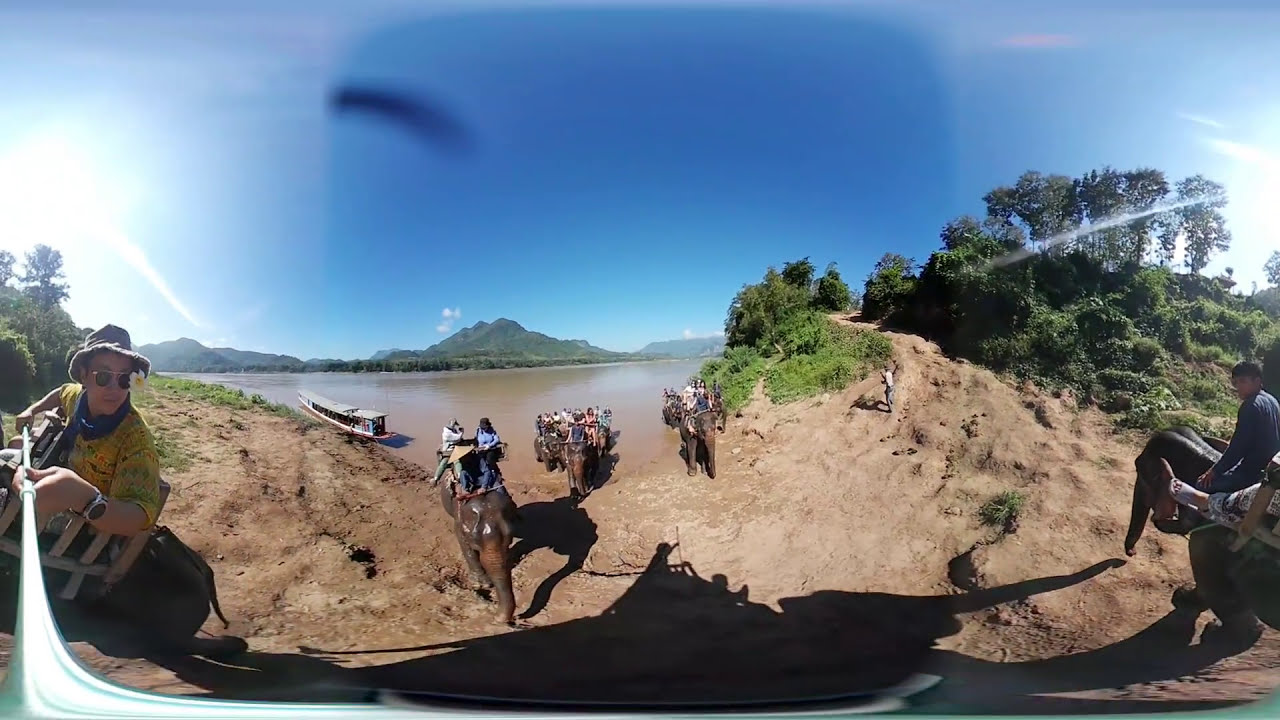In this highly detailed, panoramic outdoor image, a group of tourists is riding majestic elephants amidst a serene landscape. The rectangular, possibly VR or 360-degree photograph captures various people on top of large elephants. These elephants are emerging from a brown, water-filled river and making their way toward a sandy, tan shore, surrounded by low green bushes and trees.

On the left side, a man captures the moment with a camera while riding his elephant; he's easily identifiable by his yellow shirt, shades, and blue scarf. His extended arm holds a stick, which warps amusingly at the bottom of the photo, a characteristic of VR imaging.

In the middle of the scene, you can count four or five other elephants, each with riders donning a mix of clothing, from hats and sunglasses to cameras slung around their necks. The diversity in their attire suggests they are tourists, perhaps from different backgrounds, visiting this picturesque location.

Beyond the people and animals, the background unfolds into a green-covered landscape featuring low hills or mountains, accentuated by lush vegetation. The body of water seen earlier stretches towards these hills, creating a peaceful scene under the bright sun, which shines prominently from the upper left corner. On the right side, a dense mound of trees and bushes contrasts with the vibrant sky, completing this vibrant and immersive portrayal of an elephant expedition, likely situated in an Asian or African country.